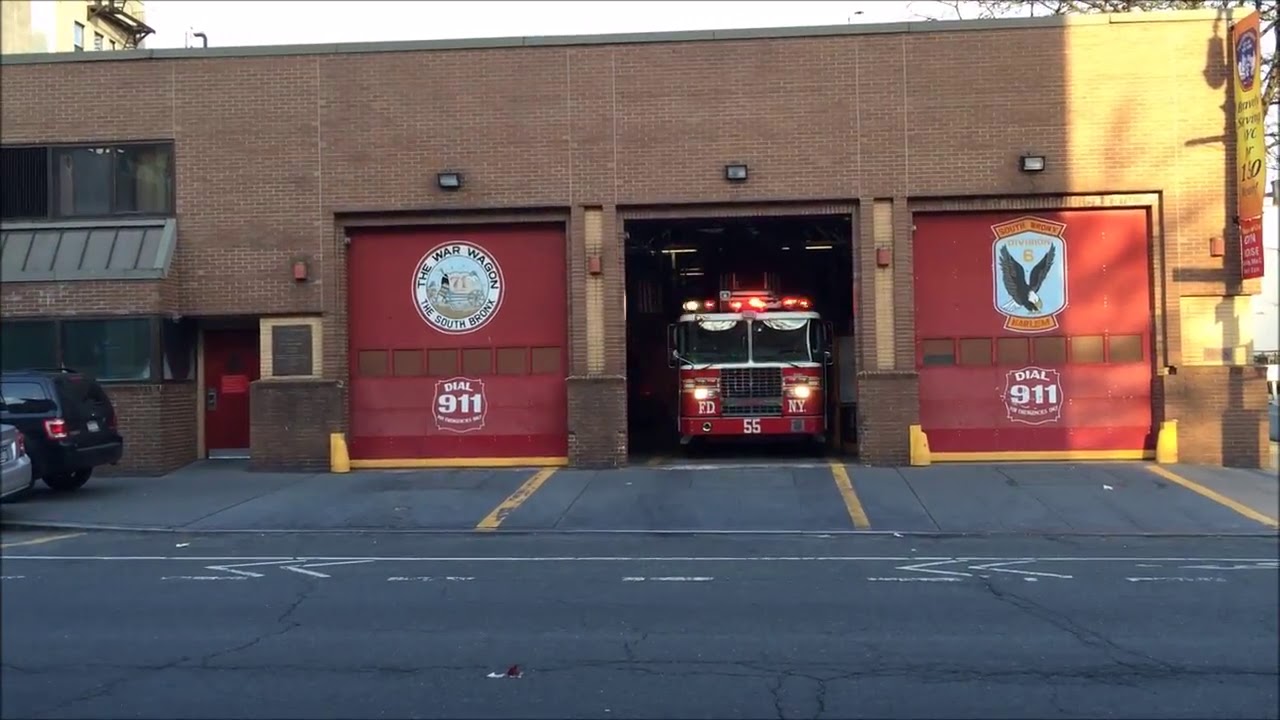This photograph depicts the front of a red brick fire station during daytime, illuminated by natural light. The building features three large red garage doors. The doors on the left and right are closed, while the center door is open, revealing the front of a fire truck with its headlights and top lights on. On the left garage door, a white circle encloses the words "The War Wagon, the South Bronx" along with an illustration of a wagon, six square windows, and a badge that says "dial 911" in white. The right garage door displays a painted badge of an eagle with "South Bronx," "6," and "Harlem" inscribed, as well as "dial 911" beneath six square windows. The fire truck, marked with "FTNY" near its headlights and the number "55" in the center, has a large square grille and windows. A banner hangs from the front of the fire station. Next to the building on the left, a red door is visible, and the back ends of two vehicles, including a black SUV, are partially seen. The area outside the station is paved with concrete and marked by yellow lines. The sky above is partly visible, suggesting overcast conditions but with sunlight clearly illuminating the station's right side.